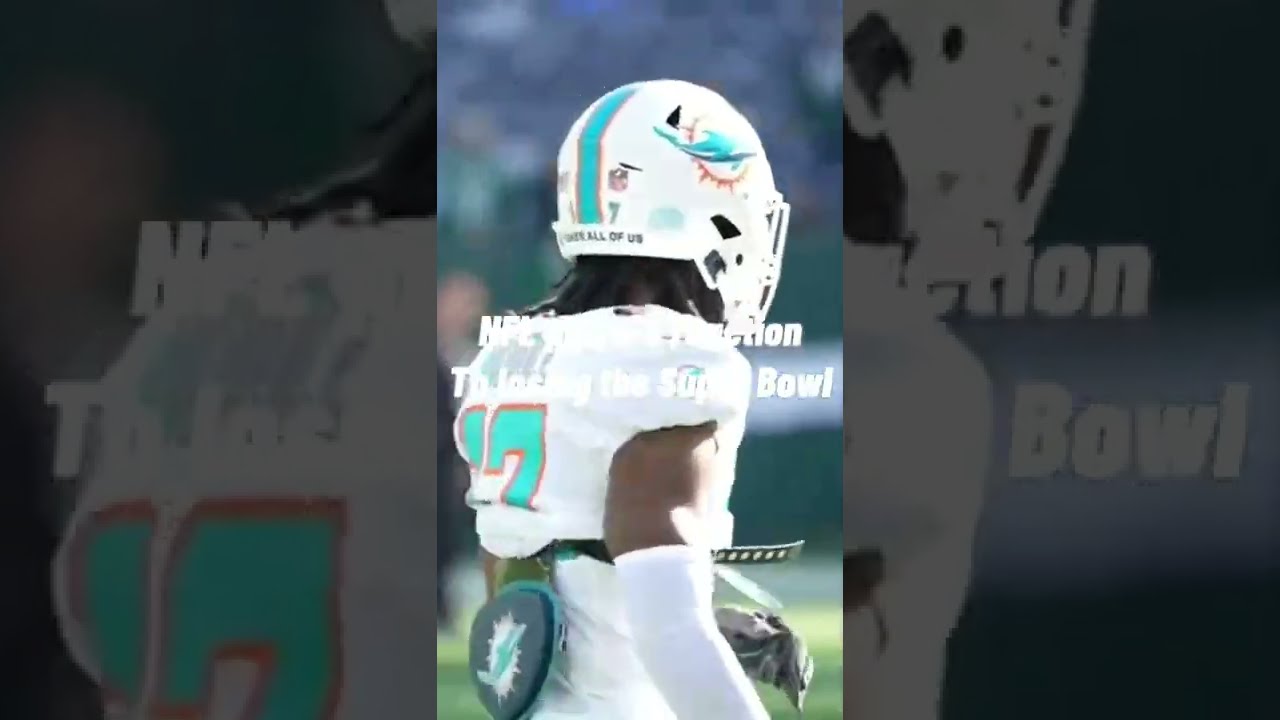The image is a horizontally rectangular, approximately six inches wide by three inches tall, and divided into three vertical sections. The narrow, colored center section features a professional football player from the Miami Dolphins walking towards the right side, with his back and right side visible. The player, who has brown skin and long black dreadlocks emerging from under his white helmet, wears a white uniform with a blue number bordered in red, possibly '17' or '27', though it’s slightly obscured. The helmet sports a blue vertical stripe and a dolphin logo, while the back of the helmet displays the phrase "All of Us" in black print. A dark gray, oblong pad with a dolphin logo is attached to the player's lower back. Visible white print across the center image includes "NFL" and partially decipherable text suggesting a connection to the Super Bowl. The blurred left and right sections magnify and darken parts of the player, emphasizing the intense contrast and focus of the central figure against the indistinct, likely stadium setting of the background.